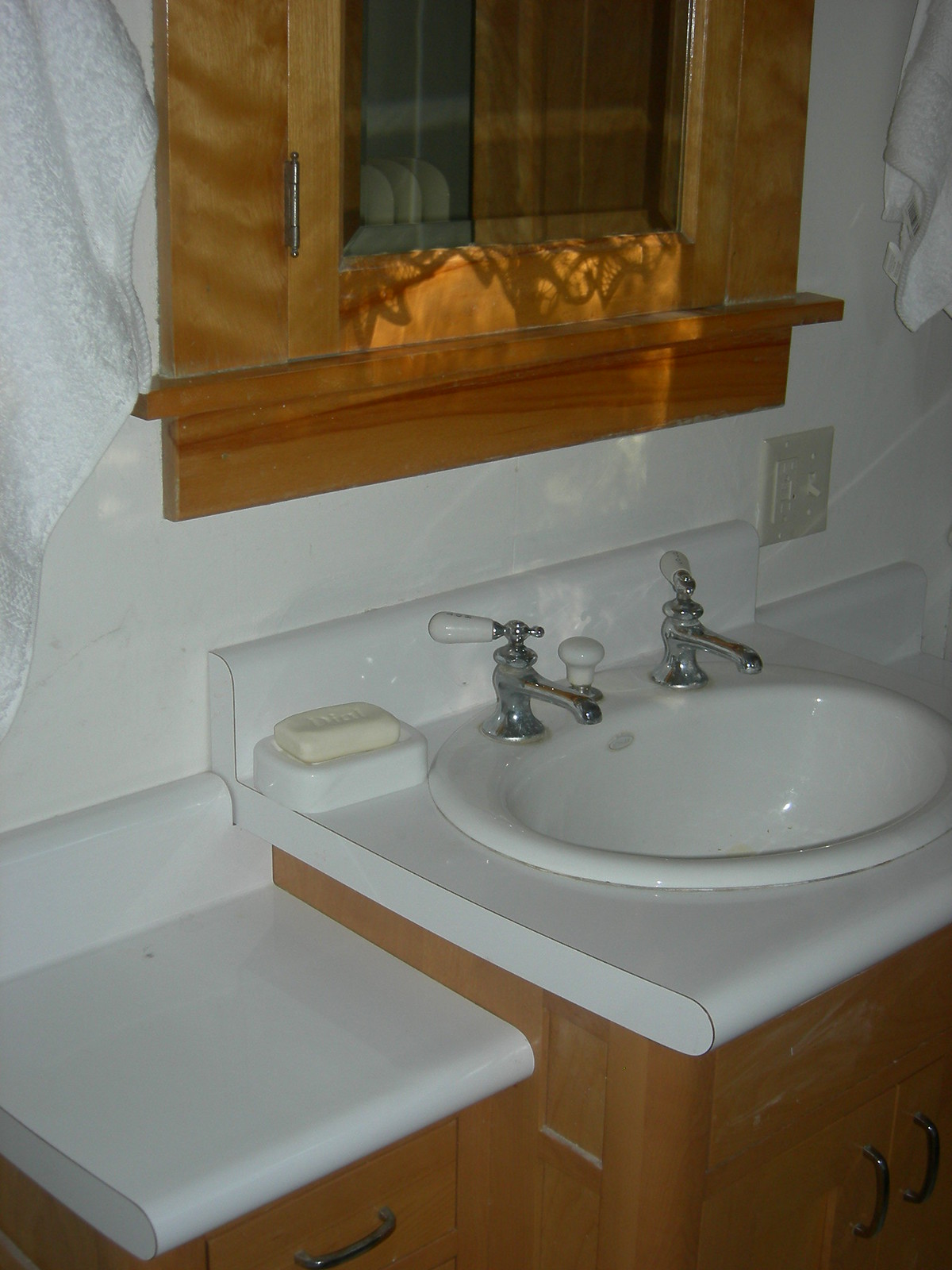The image captures a detailed section of a bathroom featuring a sophisticated design. The wall has a whitish-gray marbled finish, providing an elegant backdrop. Prominently displayed is a wooden medicine cabinet mounted on the wall; its central section appears to be either clear or mirrored, making it hard to discern precisely. Flanking the medicine cabinet are two white towels, one on the left and one on the right. Below the cabinet, slightly to its right, is a light switch.

The countertop is predominantly white and features a tiered design. The main section of the countertop is elevated, while two adjacent sections on the left and right are slightly lower in height but made from the same material. The integrated sink is positioned within the taller portion of the countertop. The sink, also white, is complemented by two chrome faucets with white trim.

A white soap dish holding a bar of soap is situated on the countertop. Below the vanity area, matching white cabinets are equipped with handles, providing ample storage. On the smaller, lower section of the countertop to the right, there are visible drawers, enhancing the functionality of the space.